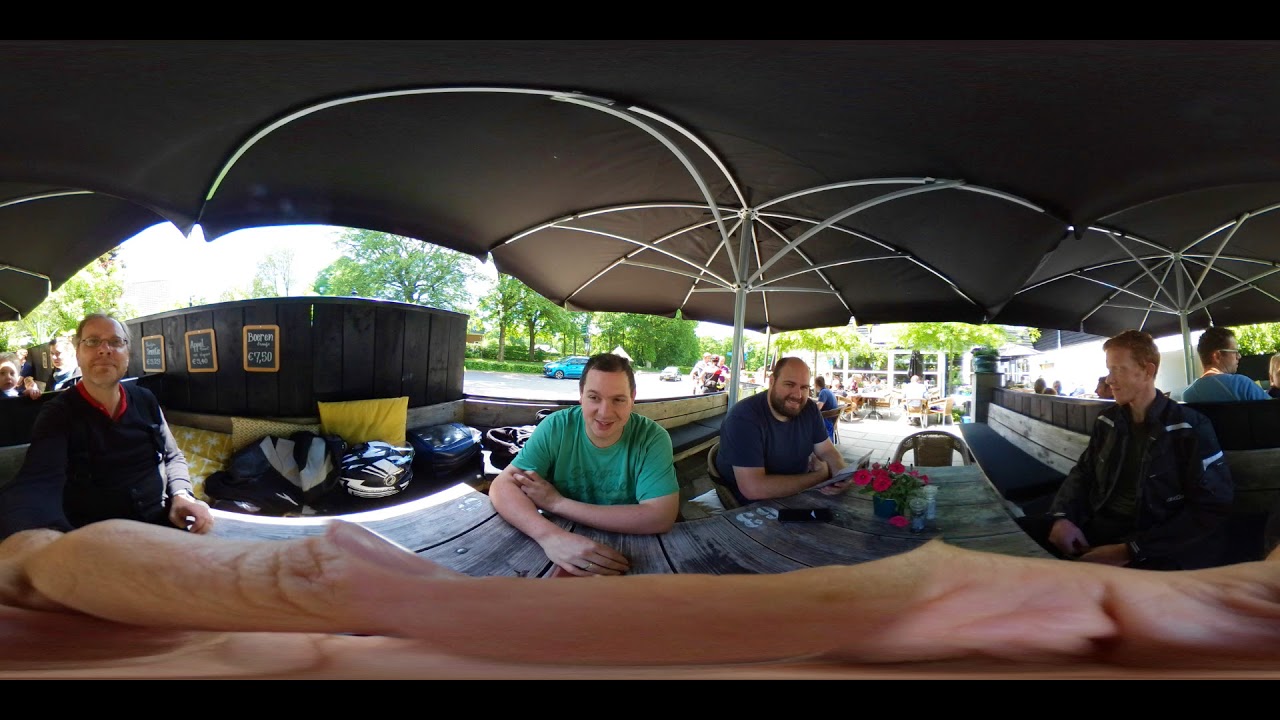The photograph captures a panoramic view of a group of people gathered under a large, black, pavilion-style canopy tent. At the top of the image, the tent's gray cover is supported by metal bars. The surroundings outside the tent are visible, including trees, cars, a street, a white metal fence, and a black building. Several people are seated at wooden picnic tables under the tent, and there's a sense of a communal gathering.

In the foreground on the left, there is a man wearing a blue top, holding a camera with his left hand. Due to the panoramic nature of the photo, his arm appears unusually elongated and stretched across the image, creating a distorted effect. Just outside the tent, to the left, there are several dark bins with labels outlined in yellow and white.

A group of men is seated at the picnic tables. Closest to the man with the camera is a man wearing a green short-sleeved shirt, with his right hand resting on the table and his left hand on his right arm. Next to him is a bearded man in a blue short-sleeved shirt with short hair, who also has his arms on the table. To his right is a man wearing a blue jacket, looking to the left, with short brown hair and his hands resting in his lap. He appears to be sitting on a bench that extends towards the rear of the tent. Behind and to the right of him, other people are engaged in conversations.

The lighting in the image indicates it is daytime, with light peeking through under the umbrellas and the edges of the tent. The background scenery includes additional walkways, cars, and structures, providing a detailed and busy backdrop to the gathering under the tent.